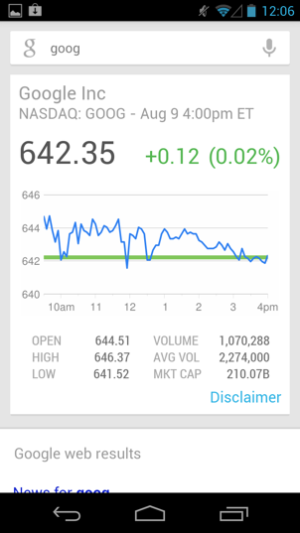Screenshot showing a stock trading app interface on a gray background with a black bar at the top. The time displayed is 12:06, and there is a cursive "G" followed by "GOOG" and a microphone icon to the right. The text "Google Inc. NASDAQ: GOOG" is prominently displayed. Below that, the current stock price is listed as $642.35, indicating a +0.12 (+0.02%) increase. 

A detailed chart at the bottom shows the stock’s performance throughout the day, marked by time intervals at 10 a.m., 11 a.m., 12 p.m., 1 p.m., 2 p.m., 3 p.m., and 4 p.m. A green line indicates the current price of $642, with a blue graph displaying fluctuating values that occasionally rise above the green line. The graph's ups and downs are consistent with typical trading patterns.

Key financial information includes:
- Open: $644.51
- Volume: 1,070,288
- High: $646.37
- Average Volume: 2,274,000
- Low: $641.52

Additional text indicates market capitalization information, and the board shows values at different price points: 646, 644, 642, and 640.